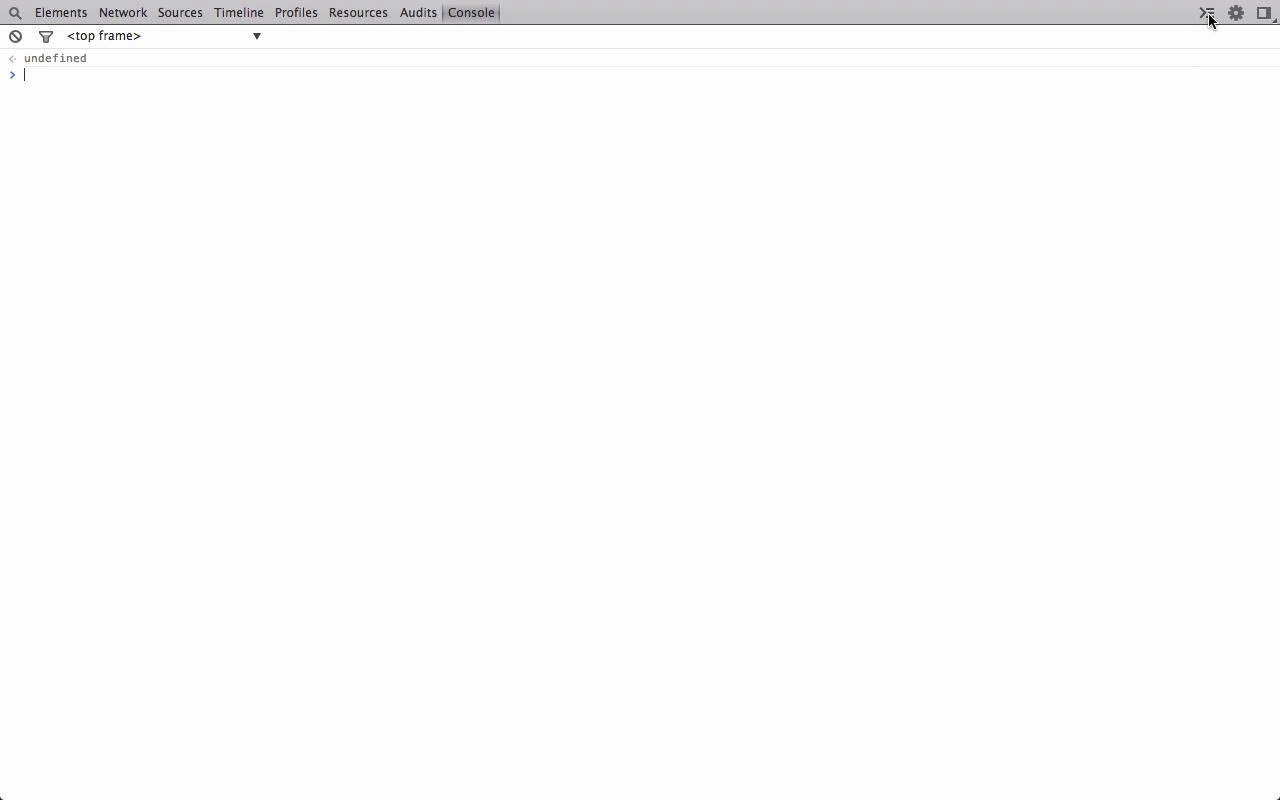The screenshot depicts a section of a computer screen, primarily showcasing the developer tools interface of a web browser. The majority of the screen is white, but at the very top, there is a medium gray navigation bar. The navigation bar includes a sequence of tabs starting from the left with a magnifying glass icon, followed by the labels: "Elements", "Network", "Sources", "Timeline", "Profiles", "Resources", "Audits", and "Console" in black font. The "Console" tab is highlighted in a slightly darker shade of gray, indicating it is currently selected. Below this, there are additional controls featuring a prohibited sign icon, a flashlight icon, and a sequence of navigational buttons including a bracketed arrow labeled "Top Frame," a back arrow, another left arrow with the word "undefined" next to it, and a blue right arrow labeled "Clicker." Additionally, a blinking cursor is visible on the screen, frozen at the moment it was captured, indicating the spot where text input is active.